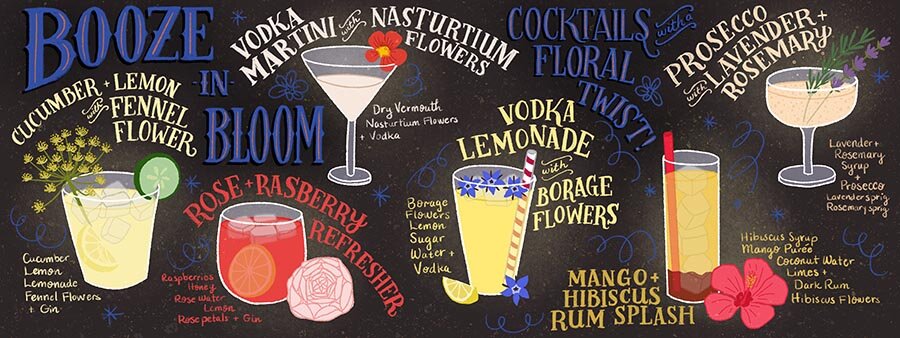The poster, titled "Booze and Bloom" in large blue letters against a black background, promotes a series of illustrated floral-themed cocktails, perfect for bars or cocktail lounges. The collection includes a variety of detailed drinks:

1. **Cucumber, Lemon, and Fennel Flowers:**
   - Served in a short yellow glass with cucumber and lemon accents.

2. **Rose Raspberry Refresher:**
   - Presented in a small, round-bottomed red glass, garnished with an orange slice and ice cubes.

3. **Vodka Martini with Nasturtium Flowers:**
   - Pouring into a martini or champagne-like glass, adorned with a red nasturtium flower on the rim.

4. **Vodka Lemonade with Borage Flowers:**
   - A clear glass filled with yellow liquid, topped with three blue borage flowers, and featuring a red and white striped straw.

5. **Mango Hibiscus Rum Splash:**
   - In a regular, slightly skinnier glass with yellow liquid, a hint of red at the bottom, and a red straw.

6. **Prosecco with Lavender and Rosemary:**
   - A larger wine or martini glass containing pink liquid, garnished with lavender flowers and rosemary sprigs.

Each drink is illustrated with ingredients laid out in vibrant colors, emphasizing both the aesthetic and the refreshing, floral nature of the cocktails.